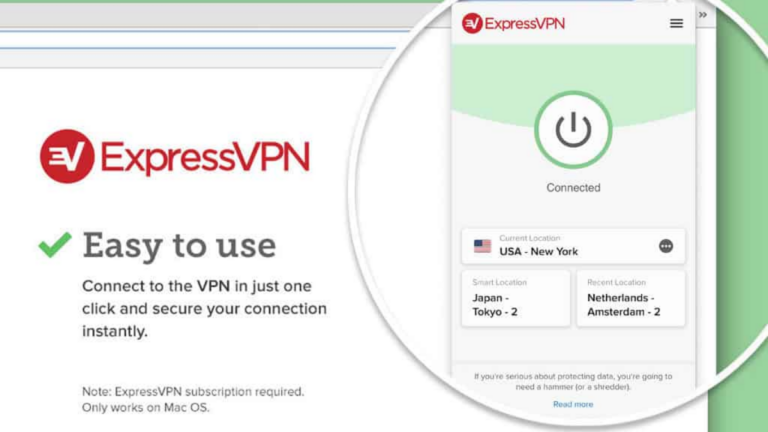This image, captured from a cell phone screen, displays a user interface for ExpressVPN. At the top, there is a prominent logo featuring a white 'V' interlinked with a backward 'E', all set within a red circle. Below the logo, ExpressVPN is written in bold red letters.

Moving down, a bright green check mark accompanies the text “Easy to Use,” indicating the simplicity of connecting to the VPN service. The text explains, “Connect to the VPN in just one click and secure your connection instantly.”

Towards the bottom of the screen, in a smaller font, there is a note: “ExpressVPN subscription required. Only works on Mac OS,” providing essential usage information.

In the upper right corner, a zoomed-in area highlights a green button with a power symbol, labeled “Connected,” suggesting that the VPN is currently active. The interface also displays a list of server locations: “U.S. - New York,” “Japan - Tokyo 2,” and “Netherlands - Amsterdam 2,” indicating various connection options available to the user.